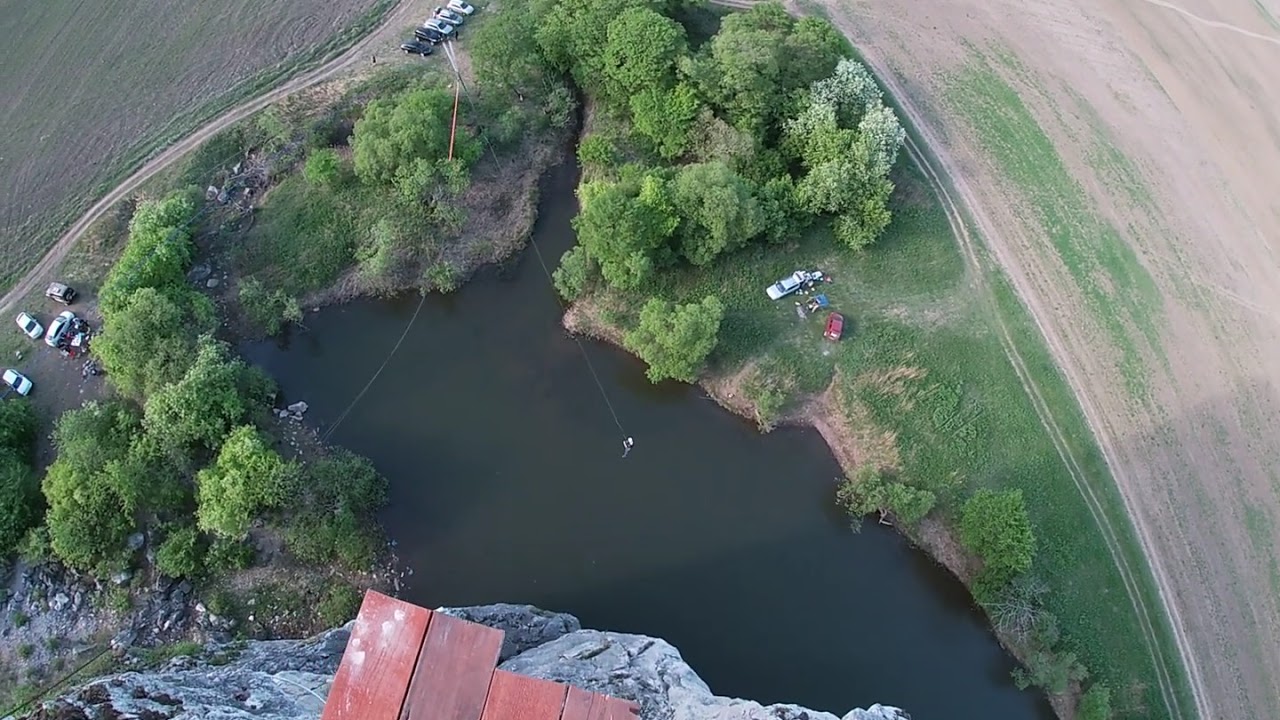The image is an aerial shot captured from a high vantage point, likely atop a mountain or cliff, offering a sweeping, detailed view of the landscape below. Dominating the foreground are four red wooden planks resting on a granite surface, which seem to serve as a jumping-off point, possibly for bungee jumping or zip-lining activities. Directly below, an irregular-shaped pond is surrounded by a mix of gray gravel and patches of green grass. Hovering over the pond is a person who appears to be either skydiving or bungee jumping, suspended with a line attached.

To the left of the pond, a strip of land encircles the water, which transitions into a densely wooded area brimming with trees. Scattered across this wooded area and the adjacent land are several cars, with around four distinctly parked on the far left of the image, and more vehicles visible in the middle left-hand side. Additionally, the green grass near these cars adds a splash of verdant color amid the natural surroundings. The entire scene is cast in the mellow light of the late evening, with the granite surface casting a long shadow stretching to the right side of the image, emphasizing the height and time of day.